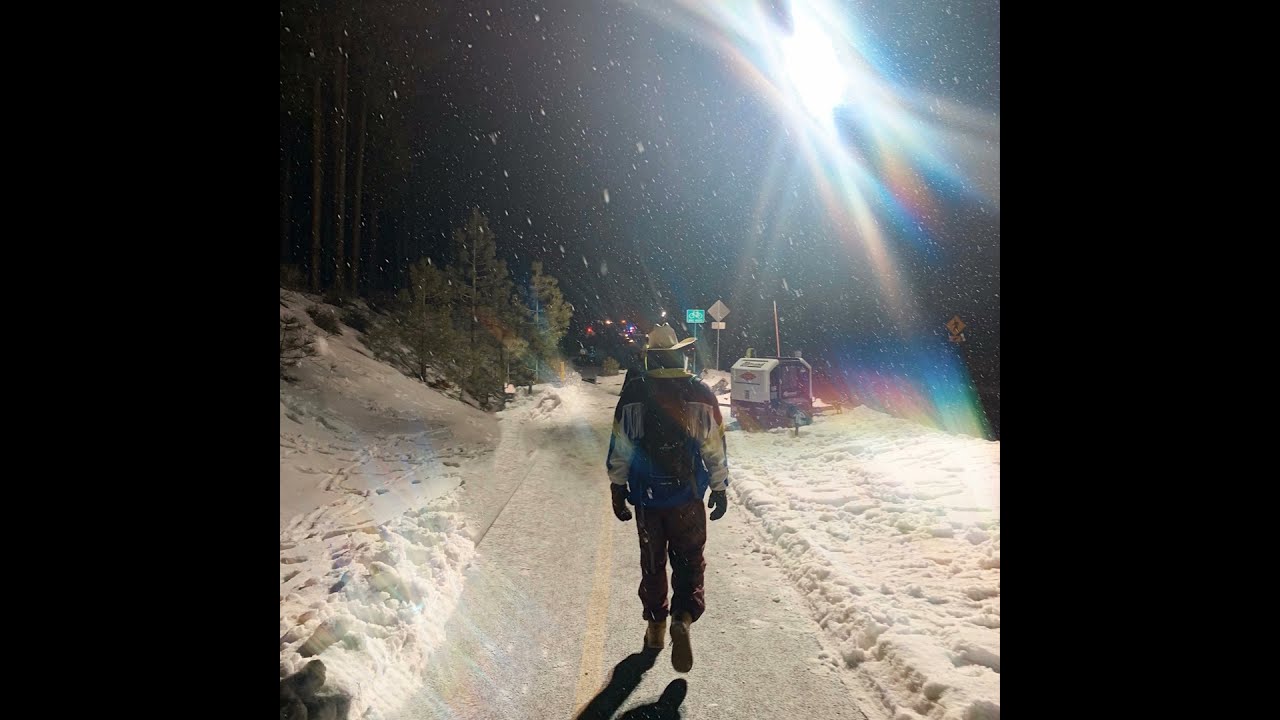In this nighttime image, we see a solitary figure with their back to the viewer, walking down a narrow, snow-covered path. The person is wearing a tan cowboy hat, long sleeves, gloves, baggy pants, and boots, giving them a western appearance. The path, possibly a bike lane, is flanked by snow on both sides and features a yellow line down the center. Overhead, a bright light illuminates the scene, casting a soft glow on the falling snowflakes. The sky is dark but blurred with what appears to be a subtle rainbow effect near the light source on the top left of the image. In the distance, trees are visible, along with faint outlines of buildings and road signs, including a green bicycle sign. The stark contrast between the dark surroundings and the illuminated path creates a serene, almost magical atmosphere.